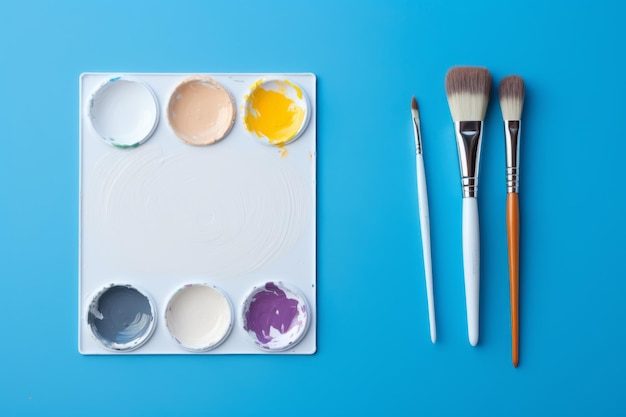The image captures an overhead view of a painting set placed on a medium blue background. Prominently, there are three paintbrushes and a white plastic paint palette. The paint palette is centrally positioned and features three circular wells on the top and three on the bottom. The top row holds white paint in the first well, a peachy-brown shade in the second, and yellow in the third. The bottom row contains a bluish-gray color in the first well, white in the middle, and purple in the third well.

To the right of the palette, three paintbrushes are meticulously arranged. The brush on the far left is small with a very light blue handle and a tiny, white-tipped bristle section that is slightly browned. The middle brush also has a blue handle but features broader white bristles, again tinged with brown near the edges. The third and rightmost brush stands out with its orange handle and slightly broad, white-bristle tip. All the brushes share a common characteristic: a shiny, chrome-colored metal section connecting the handle to the bristles.